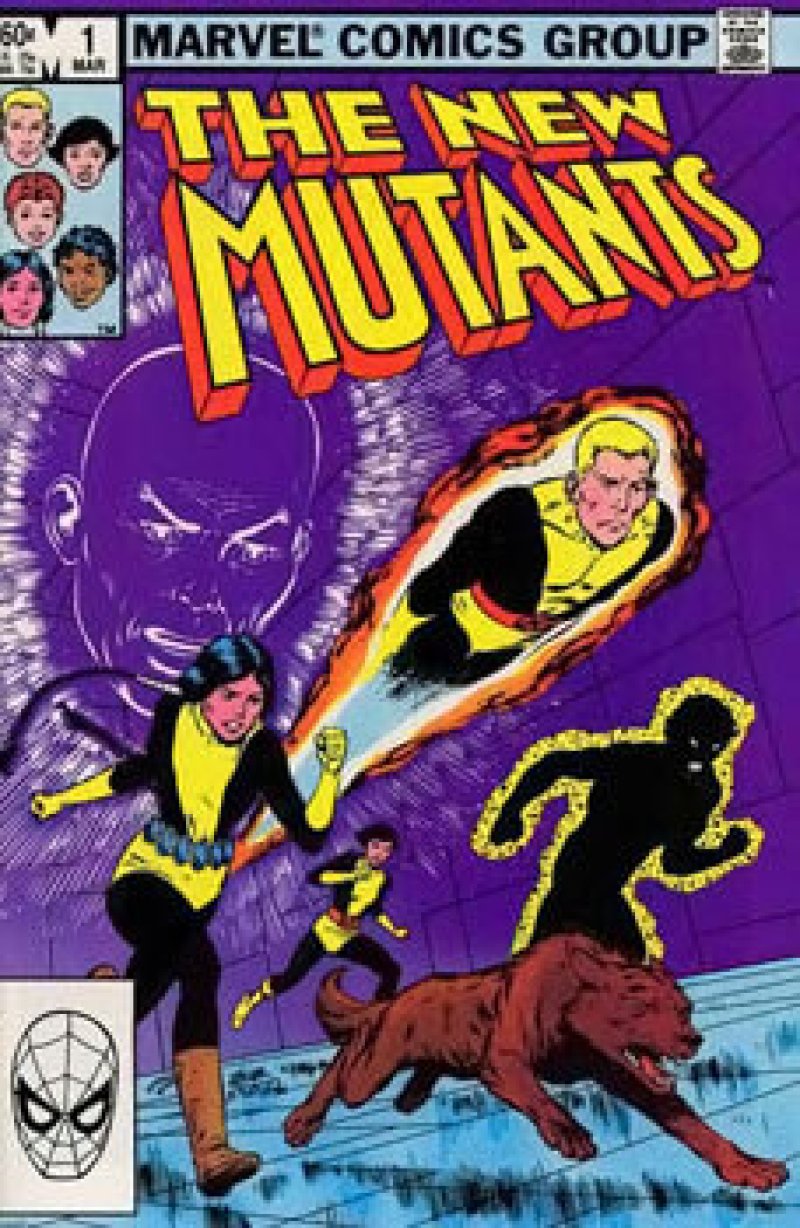The cover of the comic book is titled "The New Mutants" and prominently features dynamic artwork framed in a blue bar with black text at the top, saying "Marvel Comics Group." The book, priced at sixty cents, includes a small black and white drawing of Spider-Man's face in the bottom left corner. The title "The New Mutants" stands out in a bold, 3D effect with yellow lettering and orange edges. The main image showcases five characters in action: a white blonde man flying, surrounded by an aura; a redhead woman running; an Asian or white woman with black hair also running; a dark-skinned woman now appearing as a dark, black silhouette with a yellow glow; and a red-furred dog charging forward. Behind the group, there's a large, psychic face set against a purple background, with a bald man, possibly Professor Xavier, depicted in outline with white lights indicating telepathic powers. The characters are all dressed in black and yellow costumes, clearly identifiable as part of the X-Men series.